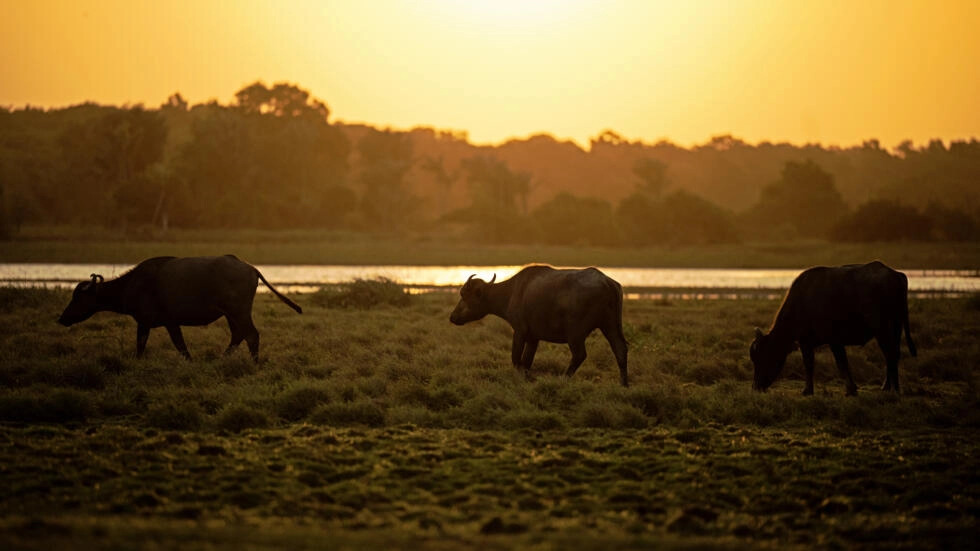This photograph captures an idyllic sunset scene featuring three cows grazing in a verdant field. The cows appear in silhouette, their dark forms standing in striking contrast against the vibrant orange sky of the setting sun. The cow on the right has its head bent down, seemingly busy eating the grass. The middle cow, distinguishable by its horns, appears to be looking forward with its head slightly lowered. The cow on the left, also facing left, has its head closer to the ground but is not actively grazing. The field varies in grass height, shorter near the bottom of the image and thicker where the cows stand. In the background, a serene river stretches horizontally across the scene, bordered by a green riverbank. Beyond that, layers of trees frame the horizon, with taller trees on the left and shorter ones on the right. Above, the sky transitions from orange to yellow hues, with a lighter, almost white area in the center, hinting at the sun's recent descent beyond the frame.